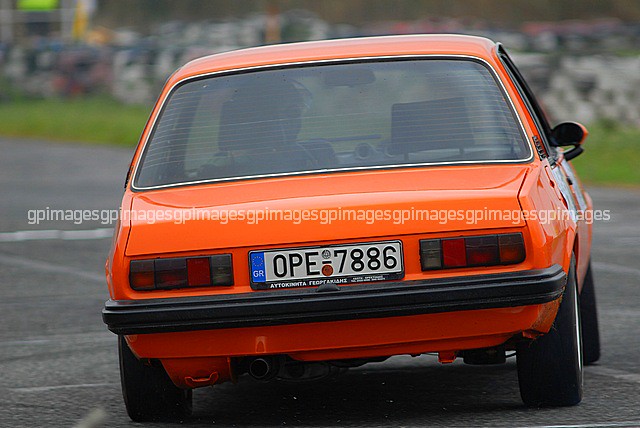The image captures a vivid orange European 1970s two-door sedan navigating a sharp left turn on a race track. The car is adorned with black rubber seals around its windows, chrome trim, and a black bumper strip, enhancing its vintage aesthetic. Notable features include red rectangular taillights and a distinct white license plate with the registration "OPE-7886." Below the license plate, there is some indistinct, likely foreign, text. The back window is decorated with fine white stripes. The track itself is paved and accented with silvery white lines, with a wide grass strip running towards a nearby safety wall. The blurred background suggests a group of spectators possibly watching from stands, indicated by a bokeh effect. The image is overlaid with the watermark "GP images" repeatedly, identifying the photographer or the image host.